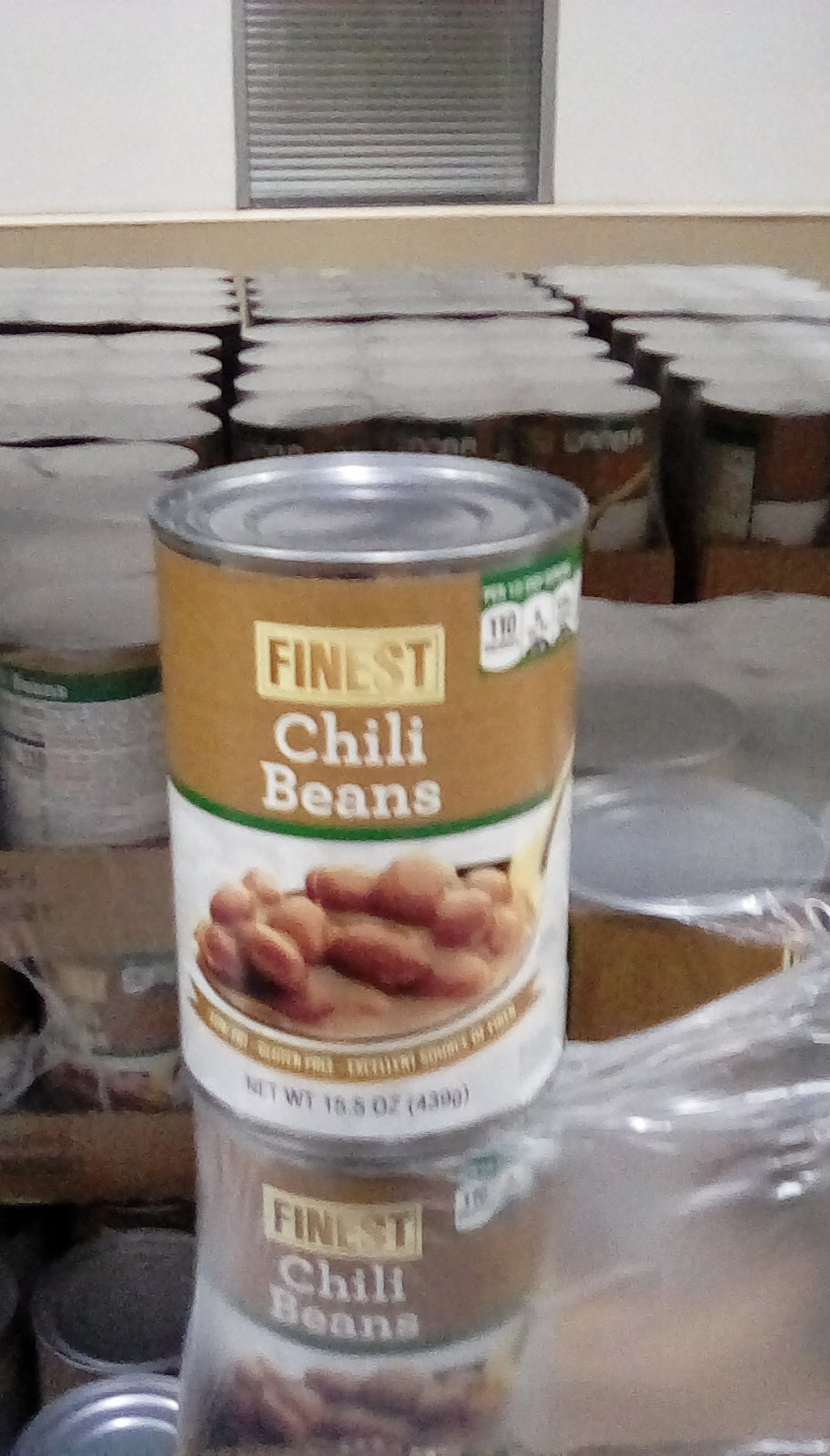This detailed photo showcases a large crate filled with stacked pallets of canned chili beans. Each pallet neatly holds 12 cans, though the exact total number of cans in the entire crate remains uncertain. The cans are branded as "Finest" and feature a label with an upper half that is a tan brownish color, while the lower half is white. Adorning the label is an image of a spoon lifting beans drenched in sauce. The additional text on the cans is blurry and unreadable. One can has been removed from its sealed 12-can pallet and is prominently displayed on top of the stack.